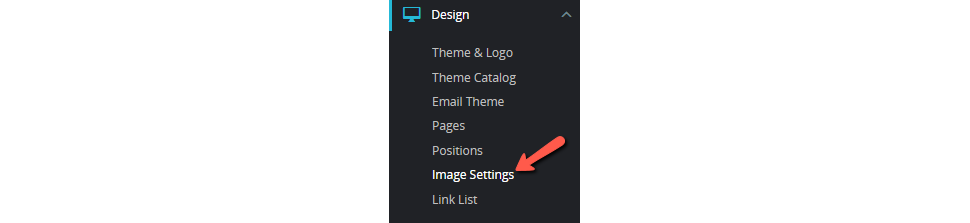In this image, there is a black square box featuring a minimalistic design. In the top left corner, there is an icon resembling a computer monitor or a TV screen, outlined with a light blue border. Next to the icon, the word "Design" is prominently displayed in white letters, and to the far right of the word, there is an upward-pointing arrow.

Below the word "Design," a menu list appears in white letters. The items in the list are as follows: 
1. **Theme and Logo**
2. **Theme Catalog**
3. **Email Theme**
4. **Pages**
5. **Positions**
6. **Image Settings** (This particular entry is highlighted in bold white letters and appears to have a slight shine. Additionally, a red arrow points directly at the final 'S' in "Settings.")
7. **Linked List**

All items in the menu, except for "Image Settings," are in a standard white font. The "Image Settings" entry stands out due to its brighter, bolder appearance and the accompanying red arrow.

The black square has a subtle, uneven border. Most of the border is consistently black, except for a small section in the top left corner where a light blue border is visible. This gives the impression that the borders are slightly misaligned.